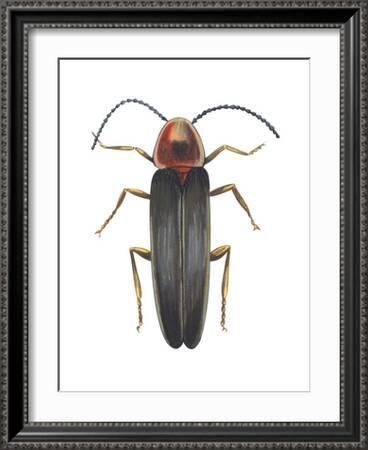This detailed illustration captures a particular insect, likely a beetle or roach, meticulously rendered by the artist and presented within an ornate black frame. The frame features detailed decorations and surrounds a clean, white mat, contrasting sharply with the white background of the painting itself. The depicted insect has a distinctive appearance with a copper-colored, oblong head adorned with two segmented, curvy antennae. The insect boasts six legs in total, varying in browns, tans, and beiges, with small fibers on their ends. Its body displays two elongated, shield-shaped wings that are predominantly black with hints of gray, covering its back. Intricate details, such as two black markings on top of the head and an overall metallic sheen, add to the lifelike representation. The insect rests in an almost aerial view, giving an impression of stillness and precision.